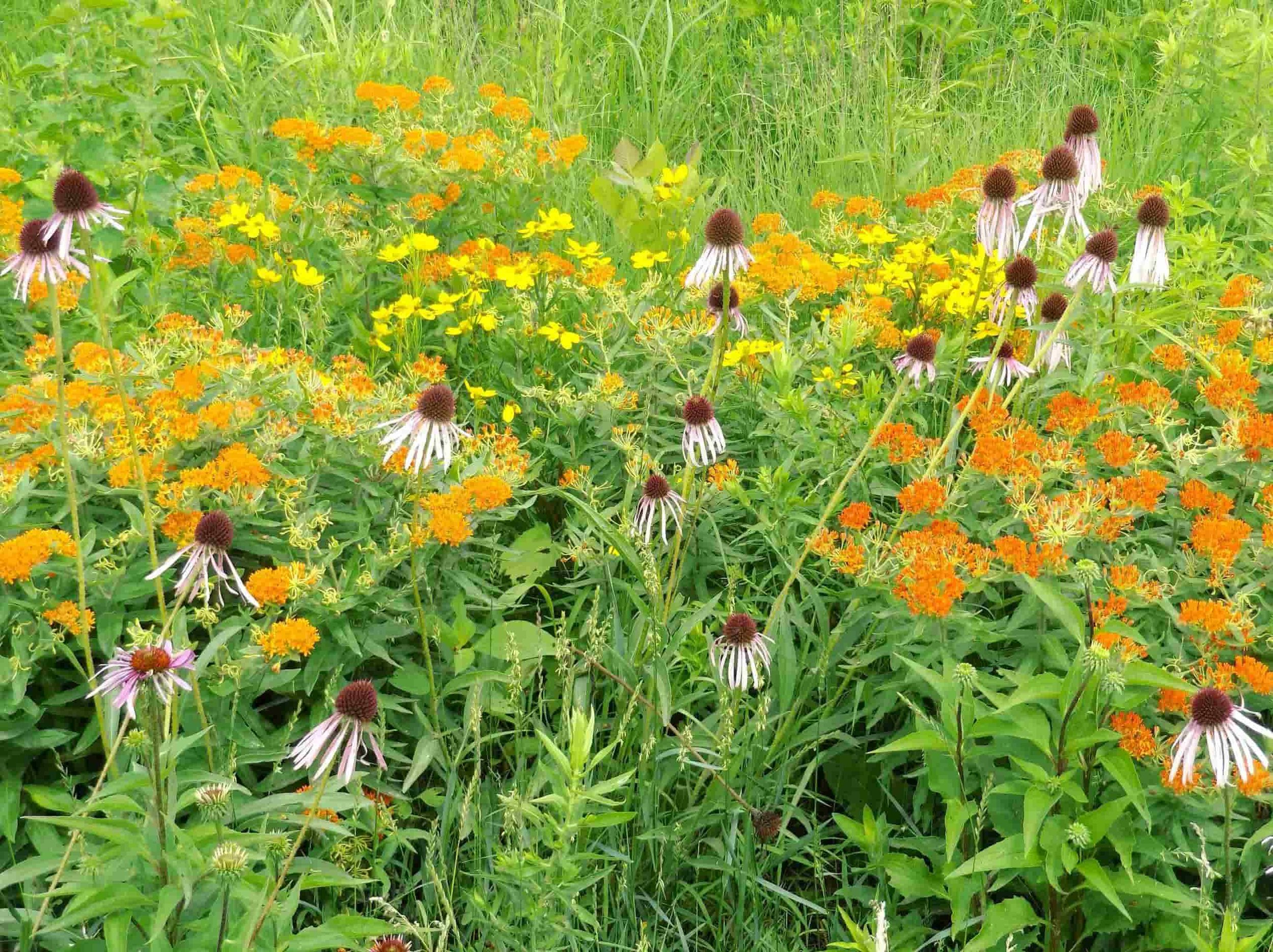The image is a vibrant, color photograph in a landscape orientation showcasing a lush, blooming field teeming with wildflowers. The scene is a harmonious blend of colors and textures, likely representing either a thoughtfully designed cottage garden or a naturally flourishing wildflower meadow. 

In the background, goldenrods and tall grasses sway gently, adding height and a golden hue to the composition. The foreground is dominated by the striking presence of echinacea, also known as purple coneflower, with their distinct rosy-purple petals radiating outwards from central cone-shaped disks. Intermingling gracefully with the echinacea are clusters of bright orange butterflyweed, also referred to as Asclepias tuberosa, bringing a fiery contrast to the ensemble.

Complementing this vivid palette are patches of yellow coreopsis, their dainty, sunlit blooms mingling among the butterflyweed. Scattered throughout the bottom right foreground, some flowers are either in the nascent stages, with unopened buds, or entering their final phase, forming seed heads—these too appear to be more echinacea. This profusion of color and form suggests a space that is both carefully curated and wildly organic, painting a picture of natural beauty at its peak bloom.